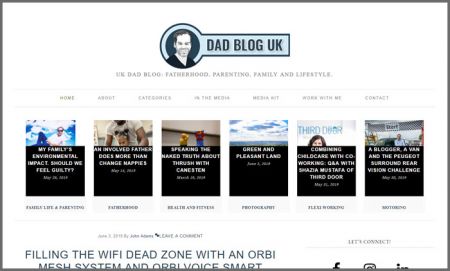Screenshot of a computer screen displaying a blog titled "Dad Blog UK." Below the title, subheadings read "Fatherhood, Parenting, Family, and Literature." A navigation menu beneath these subheadings lists six clickable options: Home, About, (the third option is unclear), and three more links—none of which are highlighted to indicate the current selection. The screen shows six images arranged in a horizontal row, each accompanied by descriptions that likely represent blog posts or articles. Below these images, an advertisement is visible, promoting the Orbi Mesh System, noted as "Filling the WiFi Dead Zone with an Orbi Mesh System" along with a mention of "Voice Smart." The blog features a white background with text and elements in various shades of gray, while the images add a splash of color. The header, resembling a key, includes the blog title on the right and a picture of a dad on the left.